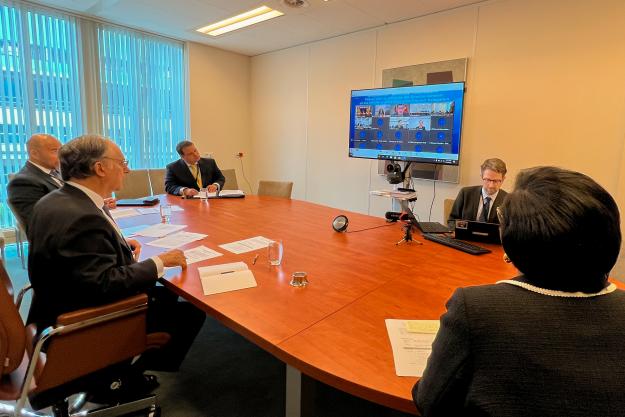In this horizontal, rectangular photograph of a boardroom, five people are seated around a large, rounded, orangish-brown table, most likely made of faux wood. Four of the individuals are men, each dressed in business suits, and the fifth person, a woman whose back is turned, sits at the far end of the table. The woman, possibly in a dress and wearing a large earring, has short, slightly rounded hair, and appears to be wearing glasses. Scattered in front of the individuals are various papers, indicative of a formal meeting. One man, perhaps the CEO, is seated alone on one side of the table. The room features peach-colored walls, a white ceiling with warm-colored strip lights, and a window to the left with partially closed curtains, obscuring the outside view. On the wall behind the woman, there is a television monitor, presumably displaying slides relevant to the discussion.